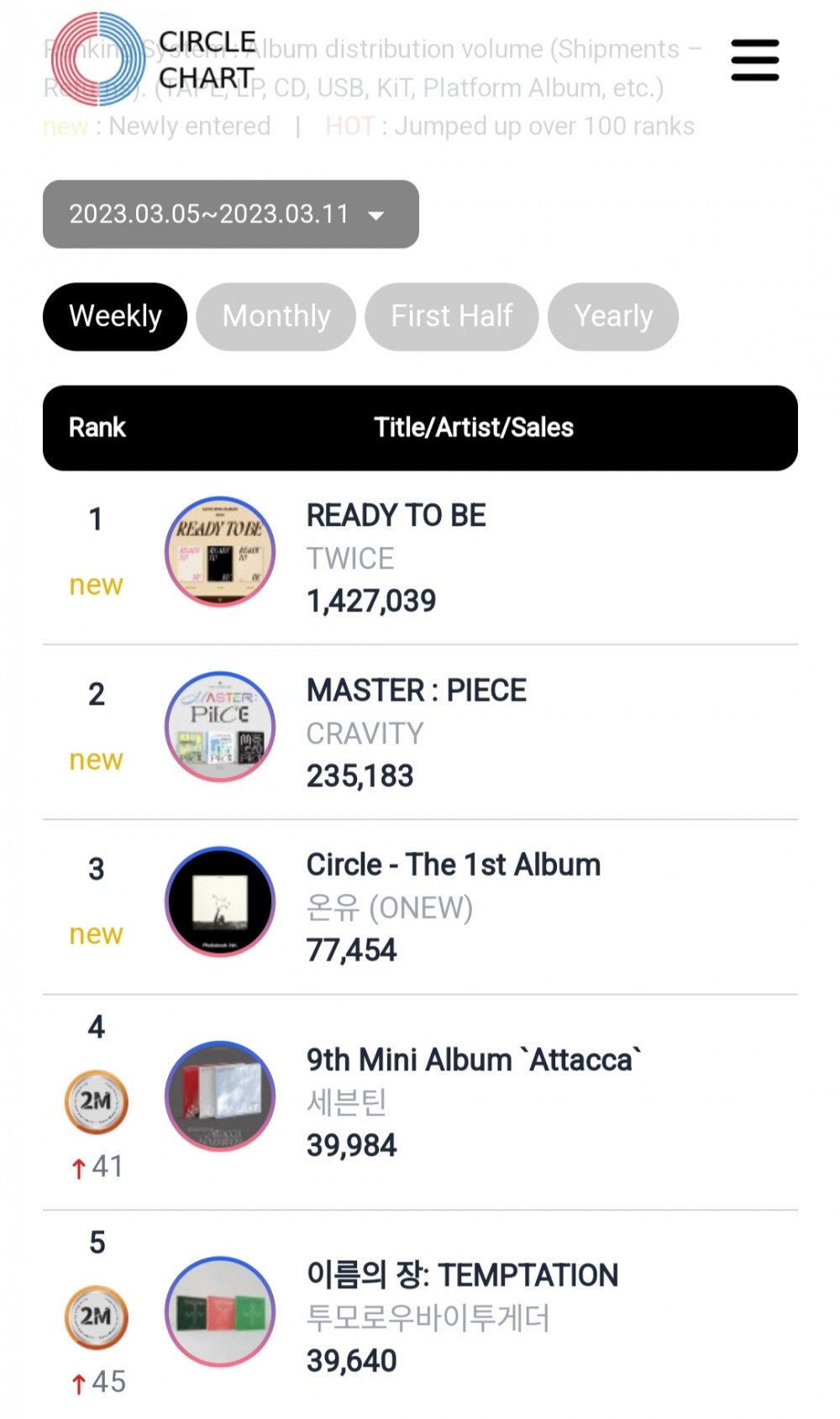This image features a screenshot of a mobile application displaying a "Circle Chart" in the top left corner. The circle is divided into two sections: one half is red, and the other half is blue. Below the circle is a bar indicating the date range "2023.03.05 to 2023.03.11," accompanied by a drop-down triangle that allows users to select different date ranges.

The app ranks various titles, artists, and sales on the platform. Five entries are listed, with the top three marked as "NEW" in yellow. The top-ranking item is "Ready to Be" by TWICE. Each title and artist pairing is accompanied by a corresponding circular photo.

The primary background color of the app is white, while the text and some bars are displayed in black. This clean, minimalist design allows for easy readability and helps users quickly discern the information presented.